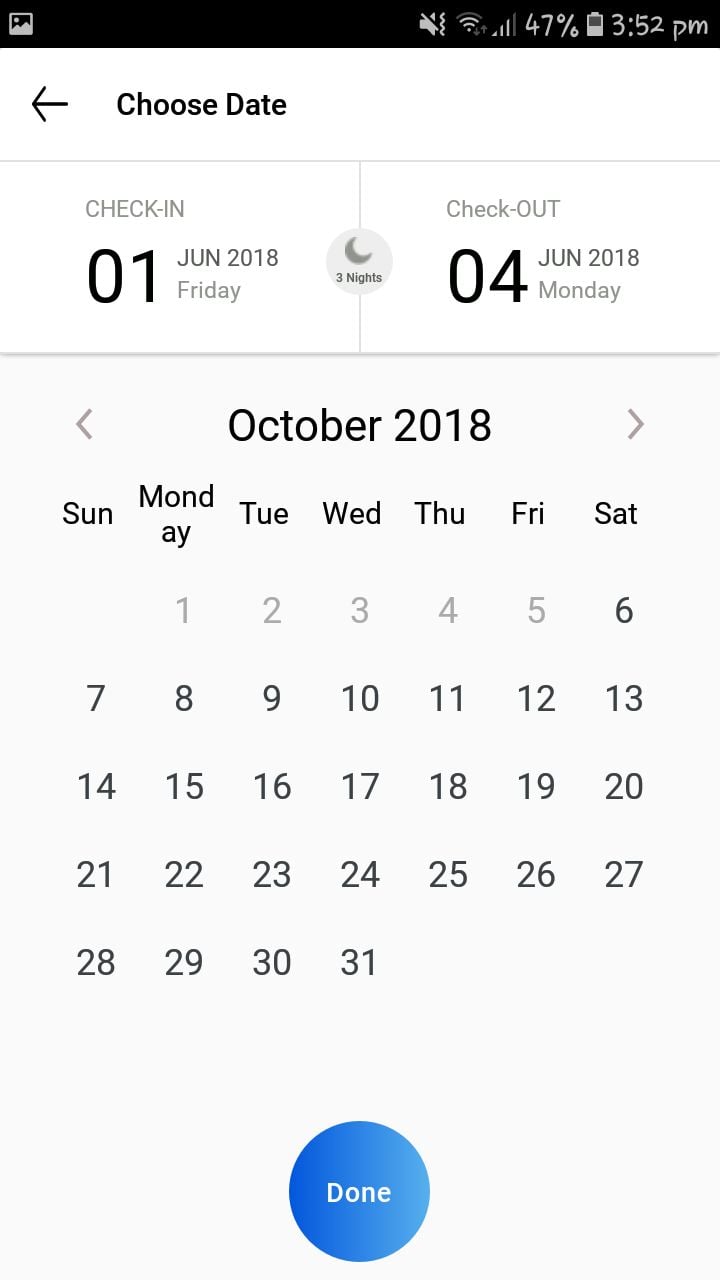A screenshot of a calendar interface within a mobile application is depicted. The upper part of the screen showcases a black bar, containing essential icons. In the upper left corner, a small image icon is displayed, while the upper right corner hosts a no-speaker icon, Wi-Fi and data signal indicators, and a battery icon indicating a 47% charge at 3:52 p.m.

Below the black bar, set against a white background, there is a left-pointing arrow accompanied by the bold text "Choose Date." The screen is divided by a gray line into two sections. The first section highlights "Check-in: 01 June 2018, Friday" and "Check-out: 04 June 2018, Monday," indicating a three-night stay, symbolized by a moon icon.

The second section displays the calendar for October 2018, spanning from Monday, October 1st, to Wednesday, October 31st. At the bottom of the screen, a bold blue circle contains the word "Done" in white font, providing a clear action button for the user to complete their selection.